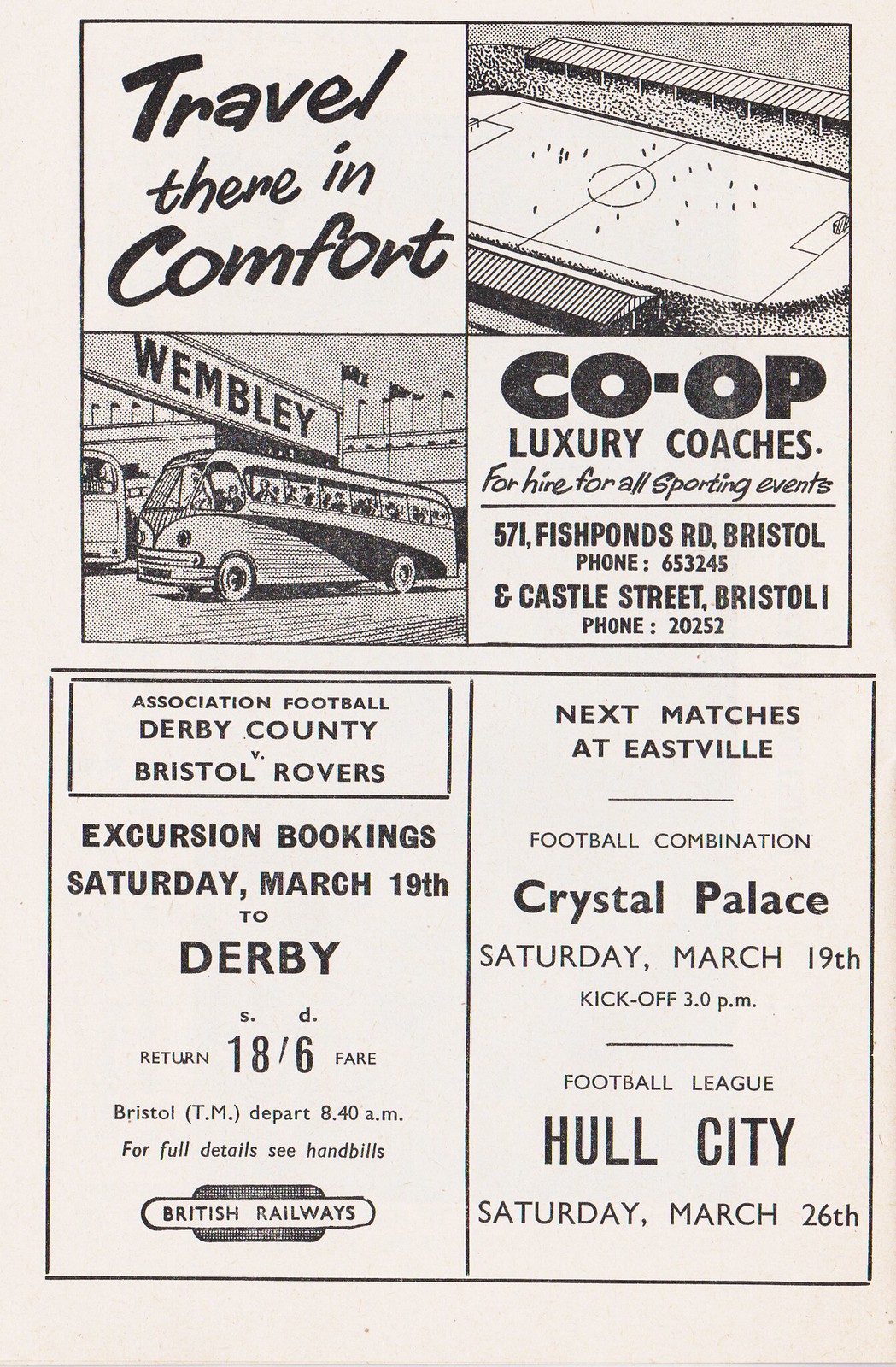A black and white, slightly sepia-toned vintage advertisement features four quadrants at the top and two rectangles at the bottom, beautifully merging imagery and text. In the upper left quadrant, the phrase "Travel There in Comfort" invites readers, overlaying a drawing of a bus marked "Wembley," filled with passengers and set against a background featuring a building adorned with flags. The upper right quadrant displays a detailed illustration of a bustling soccer stadium. Below, bold black letters proclaim, "Co-op Luxury Coaches for Hire for All Sporting Events," with contact details listed as 5571 Fish Ponds Road Bristol 1653245 and Castle Street Bristol 120252. 

The lower section contains two rectangular advertisements. The left rectangle announces an "Association Football Derby County versus Bristol Rovers Excursion Booking" scheduled for Saturday, March 19th to Derby, with a fare of 18/6 from Bristol TM departing at 8:40 AM. The bottom of this rectangle features the British Railways logo. The right rectangle informs about "Next Matches at Eastville," highlighting a Football Combination match between Crystal Palace on Saturday, March 19th at 3 PM, and a Football League match against Hull City on Saturday, March 26th.